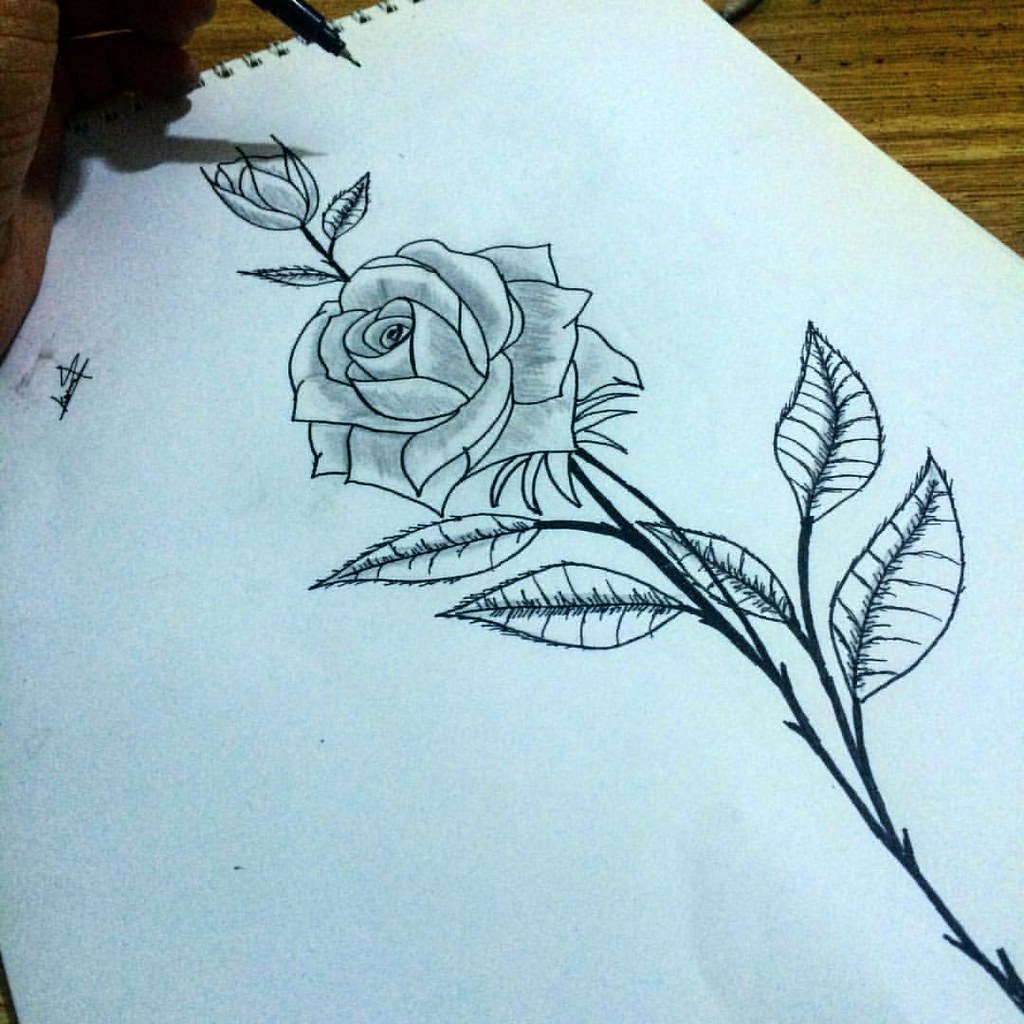This photograph, taken from a first-person perspective, captures an artist actively illustrating in a sketchbook. The artist’s left hand is visible in the top left corner of the image, with the thumb and part of the palm resting on the textured white art paper. They're holding a black pen, possibly a fine-tip or even a Sharpie, angled diagonally from the 11 o'clock position. The spiral binding of the sketchbook runs along the left short edge, indicating the paper is in landscape orientation.

The artwork features a detailed black outline of a fully bloomed rose with light shading. The petals are intricately drawn, interlocking and cascading towards a darker center, which is emphasized with fine gray hatching. The right side of the petals appears white, while the left side is shaded in dark gray, adding depth and dimension. Surrounding the rose are several leaves, each with thin black borders and vein details created using short, curved black lines. These leaves are attached to stems that start at the bottom right corner and extend off the page.

In the background, there’s a smaller, closed rosebud, shaded with the same meticulous attention to detail, and a small rose-like flower with two side leaves. Additionally, there are a few inscrutable marks that could be numbers or the artist’s signature in the top left corner. This sketch appears to be a spontaneous, yet thoughtfully executed, piece of art created during the artist's free time.